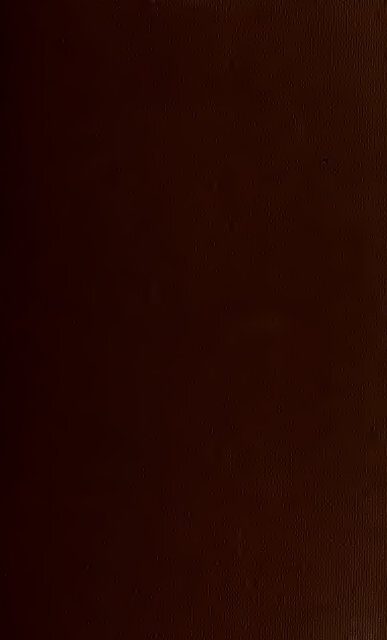The image depicts a vertically-oriented, elongated rectangular box that is predominantly black, with subtle brownish and reddish undertones. The dark rectangle is accented by some white areas positioned on both the left and right sides, and it features no discernible imagery, lettering, or figures. The background is equally nondescript, highlighting the pure blackness of the central rectangle. The monochromatic and minimalistic nature of the picture leaves little else to describe other than its stark, simple form.